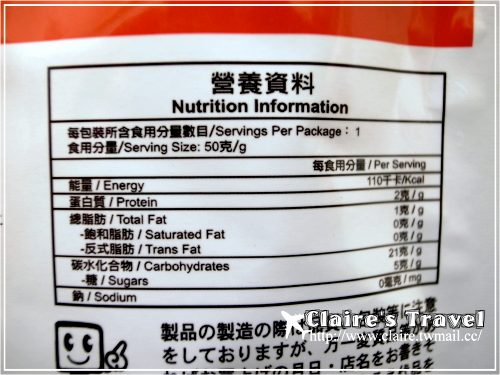This landscape-oriented photograph features a detailed shot of a nutrition label written in Chinese characters. The label is affixed to a white bag, which has a striking red bar running horizontally across its upper section. Various Chinese characters are prominently displayed throughout the label, offering nutritional information. In the bottom left corner of the image, an animated figure is depicted, pointing upwards towards the nutrition label, guiding the viewer's attention. The bottom right-hand corner of the photograph includes a watermark that reads "Claire's Travel" with a corresponding website address, claire.twmail.cc, adding a touch of professionalism and credit to the image.